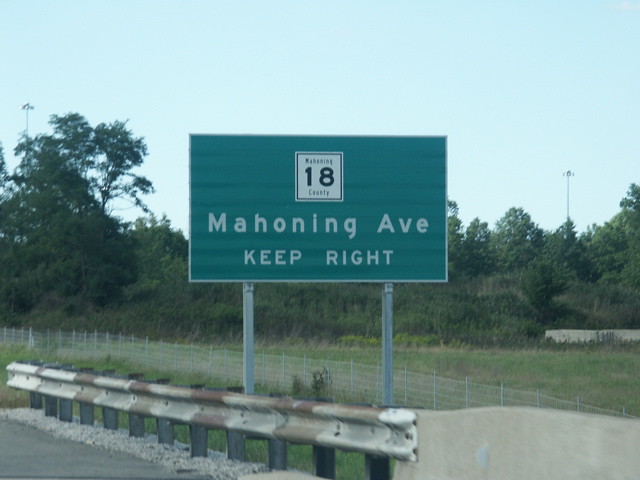In the image, a green street sign reading "Mahoning Avenue, Keep Right" and "Mahoning 18 County" in white letters prominently stands out. The sign is positioned near a small fenced area along the road, with a large gravel and white rock barrier providing protection at its base. Behind the sign, tall silver lighting structures, possibly stadium lights, are visible, adding a sense of height and distance. The backdrop is adorned with numerous trees, creating a natural boundary. There is also a grassy area near the bottom of the sign, enhancing the scenery with greenery. In the lower right corner, a cement barricade is partially visible. The photo captures a sense of motion, suggesting that it was taken by a person while driving.